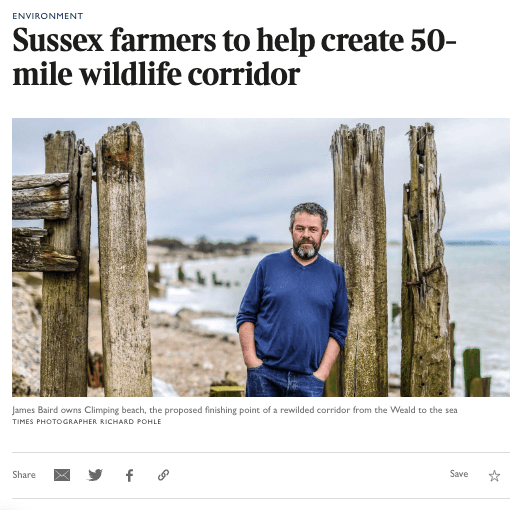The image captures an article from the environment section of a newspaper, with a headline in bold black letters that reads: "Sussex Farmers to Help Create 50-Mile Wildlife Corridor." A photograph accompanies the article, depicting a man standing beside a weathered and partially collapsed fence that is about two heads taller than him. The fence appears to form part of a wall. The man is wearing blue jeans and a blue long-sleeved V-neck shirt. He is Caucasian with a beard and mustache that have white sections, suggesting some graying. His hair is brown with streaks of gray. In the background, there is a body of water, which may be a lake or the ocean, and a sandy beach area scattered with rocks. Wooden structures extend into the water. The caption of the photograph reads: "James Baird, owner of Clipping Beach, the proposed finishing point of a rewilded corridor from the Weald to the sea. Times Photographer: Richard Profile." At the bottom of the article, it encourages readers to share it on social media.